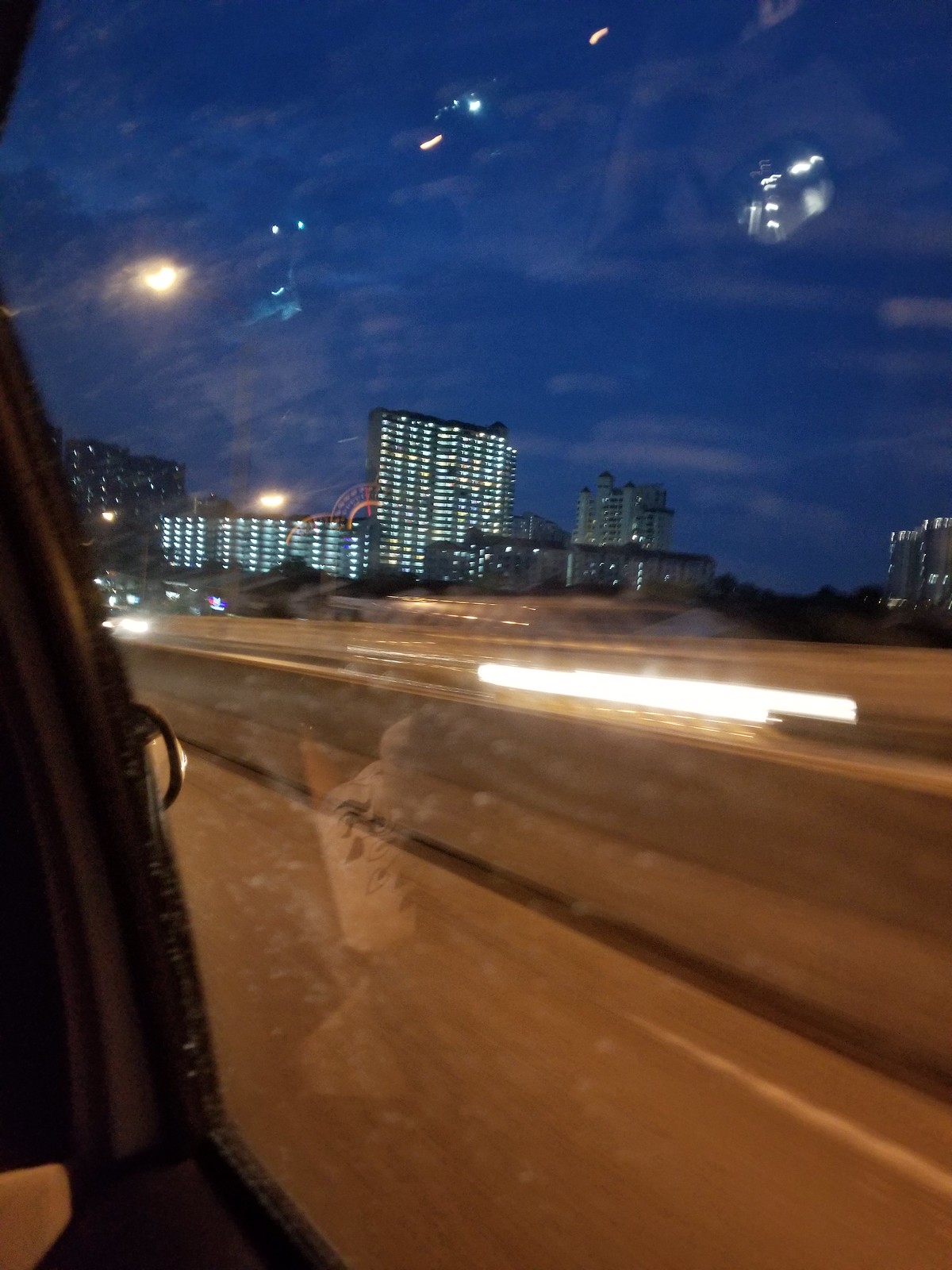Through the large blue-tinted window, possibly from a bus or airplane, we observe a detailed, reflective scene. Illuminated strip lights line the edge of a road, and a red light punctuates the scene. In the background stands a multi-story building, likely a hotel, lit up against the almost midnight-blue sky. The reflection on the window captures additional interior lights, adding to the complexity of the image.